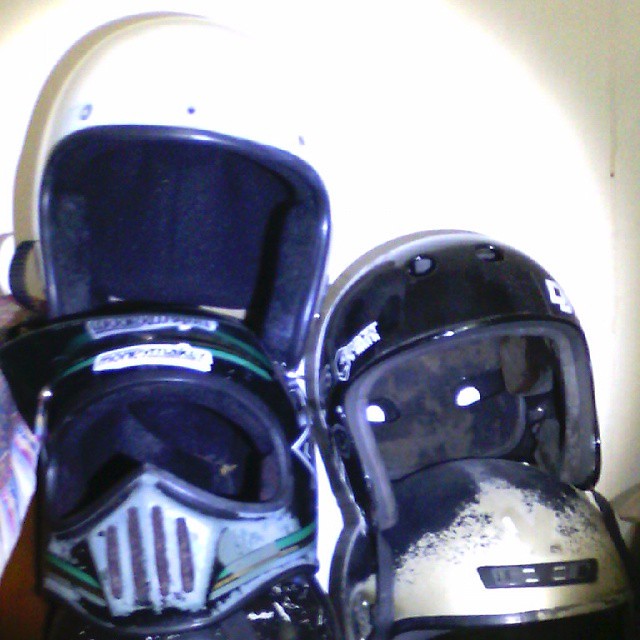The photograph features a collection of four motorcycle helmets arranged against a white wall, highlighted by a round halo-like glow from a light source behind the camera. On the far left, a fragment of a table with a blue and purple tablecloth is visible. The detailed description begins with the bottom helmet, which might be used for motocross or motorbiking, featuring an open-eye section without a shield. This helmet stands out with a metallic mouthpiece adorned with a pentagon and four red stripes, flanked by green and yellow stripes. The paint is peeling, revealing a worn look, with white branding on top. This helmet appears to rest atop another obscured helmet.

Above this, a helmet seems to be precariously tilting towards the back. On the right, there are two black helmets stacked on top of each other. The bottom helmet shows signs of wear with noticeable discoloration and a prominent white spot. Both of these black helmets lack face coverings and visors, revealing only the head and ear sections. The overall impression is one of varied, well-used helmets, each with distinct characteristics and wear patterns.